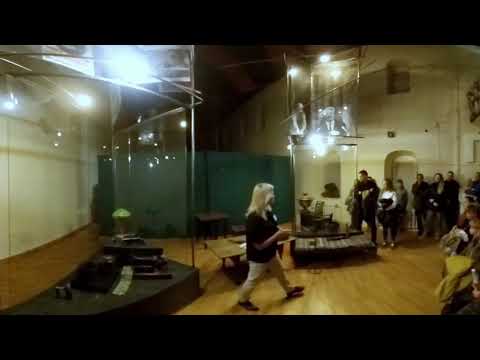The image depicts an indoor museum scene featuring various people and exhibits. On the left-hand side, there is a small black stage encased in glass, containing items such as an old-fashioned dark wood stove, a blender, and a receipt, all displayed on a wedge-shaped stand. The museum's wooden floor is visible, and in the center of the image stands a woman with long blonde hair, wearing a black shirt and beige pants, possibly a museum employee or tour guide. She appears to be either walking or giving a demonstration. Towards the right-hand side, approximately six or seven individuals clad mostly in black clothing are gathered in a semicircle, seemingly observing the woman or other exhibits. White walls and the high ceiling create a spacious backdrop for the scene.